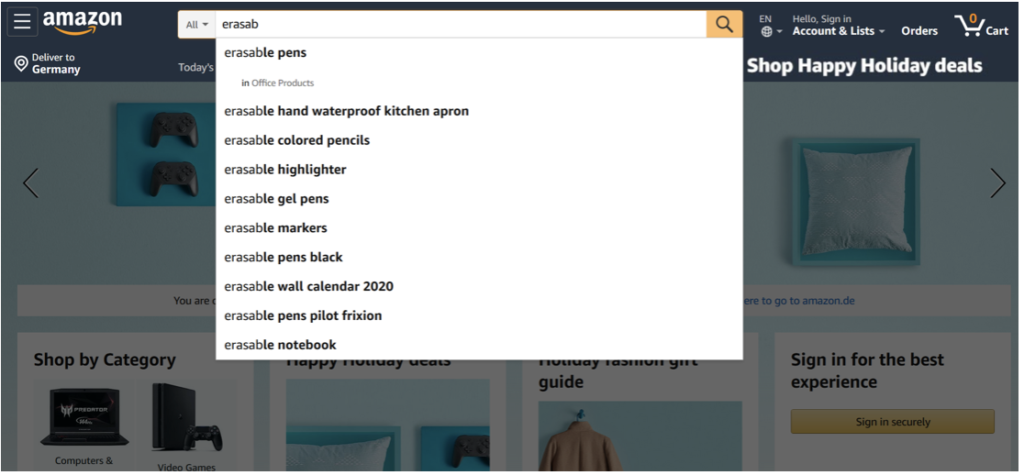The image captures a screenshot of the Amazon.com homepage during a search session. The search input field displays the partially typed query "E-R-A-S-A-B," prompting Amazon's autocomplete feature to suggest various related products. The suggestions listed include:

- Erasable pens in office products
- Erasable hand waterproof kitchen apron
- Erasable colored pencils
- Erasable highlighter
- Erasable gel pens
- Erasable markers
- Erasable pens black
- Erasable wall calendar 2020
- Erasable pens Pilot Frixion
- Erasable notebooks

Above the search bar, the site features links for "Shop Happy Holiday Deals," "Account," "Sign-In," "Orders," and "Cart," with the language setting indicated as English (EN). The top left corner displays the iconic Amazon logo, and beneath it, the delivery location is set to Germany, suggesting the user is either based in Germany or intends to send items there. Additionally, the user has not yet logged in, as shown by the invitation to "Sign-In." This detailed representation highlights Amazon's user-friendly interface and its predictive search capabilities designed to enhance the shopping experience.